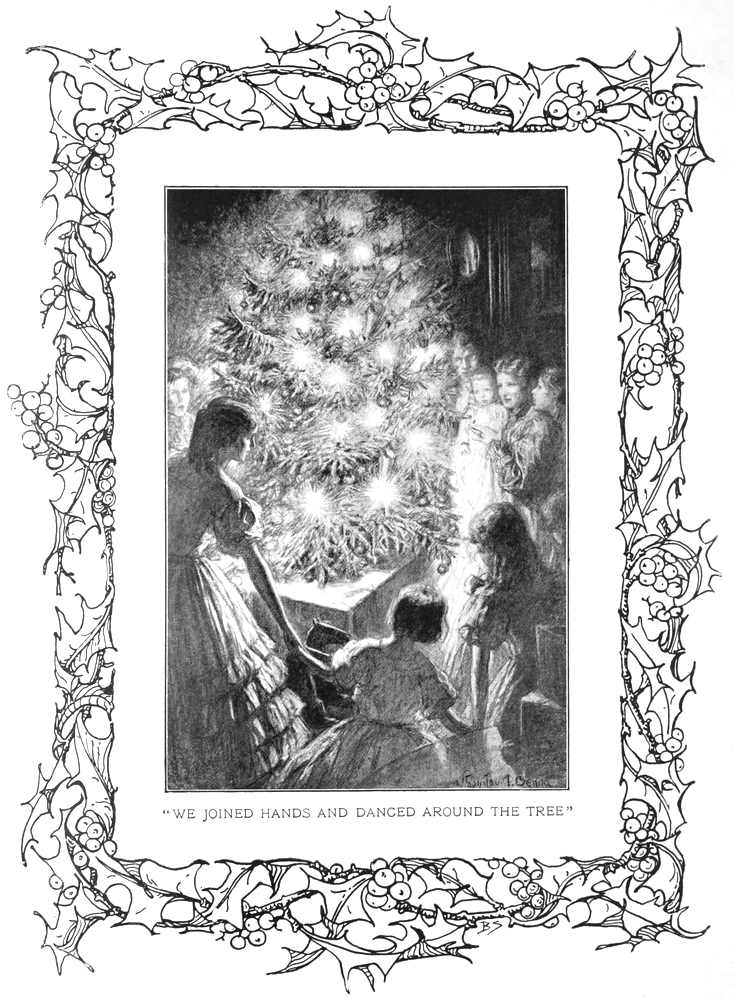The image features a digitally crafted, black-and-white holiday card centered around a nostalgic and festive scene. The centerpiece is a lit-up Christmas tree adorned with lights, placed on a table draped in a tablecloth. Surrounding the tree are three girls in the foreground, holding hands, with one gazing towards the illuminated tree. In the background, four more women, including an older woman holding a child, are all transfixed by the festive tree. The entire image is framed by an intricate embroidery pattern, typical of Christmas decorations, featuring white berries, branches, and leaves. This embroidery is colorless and traced, with the inner border highlighting a picture frame. Below the frame, black text within quotations reads, "We joined hands and danced around the tree." The lower right corner of the painting bears a small, black signature. All individuals in the image are dressed in period-appropriate dresses, enhancing the vintage Christmas ambiance.